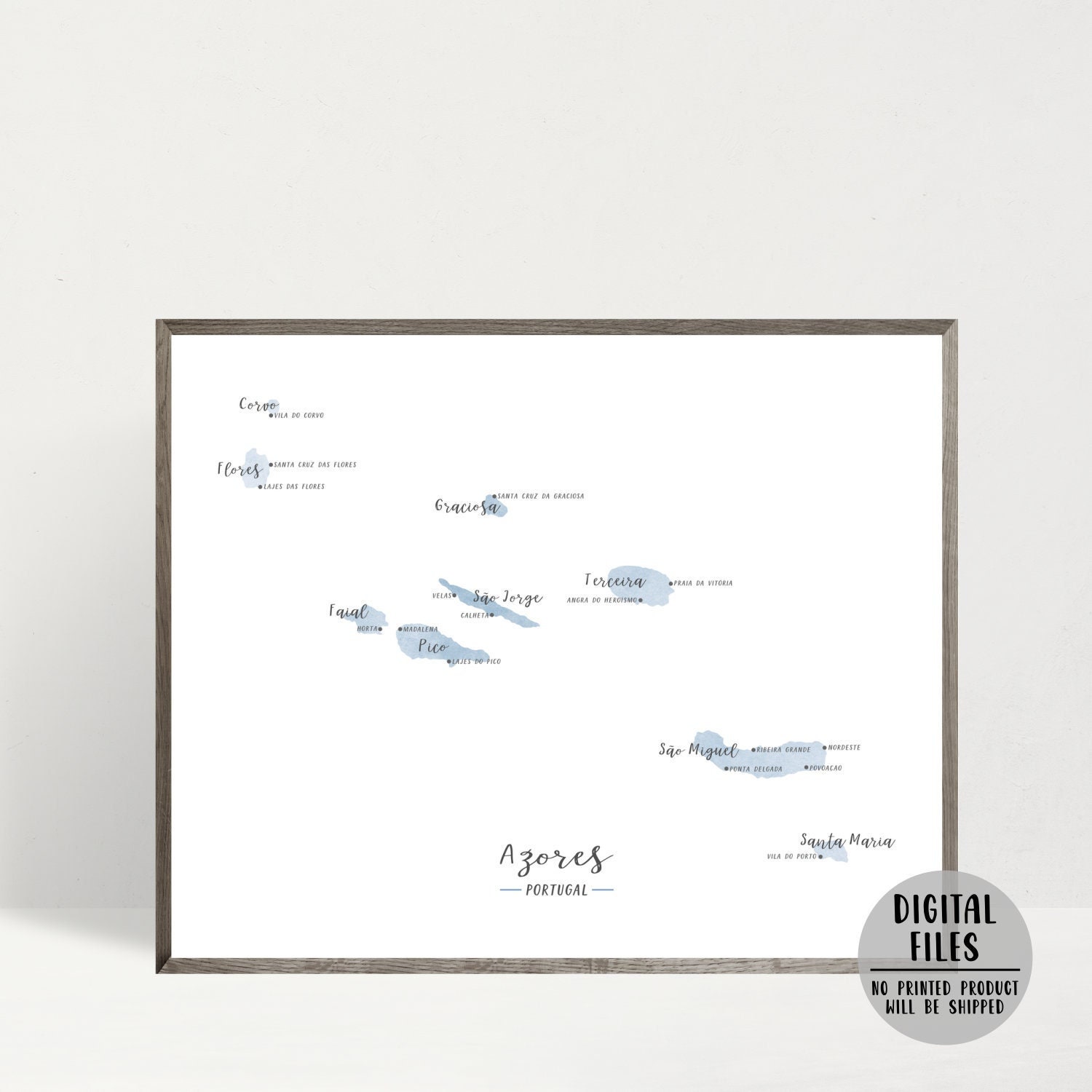This framed picture features the islands of the Azores archipelago set against a stark white background. The frame itself is thin and dark gray, likely made of wood, exhibiting a characteristic wood pattern. The artwork showcases the nine islands, depicted as variously sized, muted blue shapes, each labeled with black text in a script font. Notable islands include Corvo, São Miguel, Flores, and Pico. At the bottom of the picture, the text reads "Azores, Portugal." Additionally, the image bears a circular watermark in the lower right corner stating, "Digital Files. No Printed Product Will Be Shipped." The artwork is mounted on a white wall, casting a shadow on the lower left side, with a similarly white floor beneath.